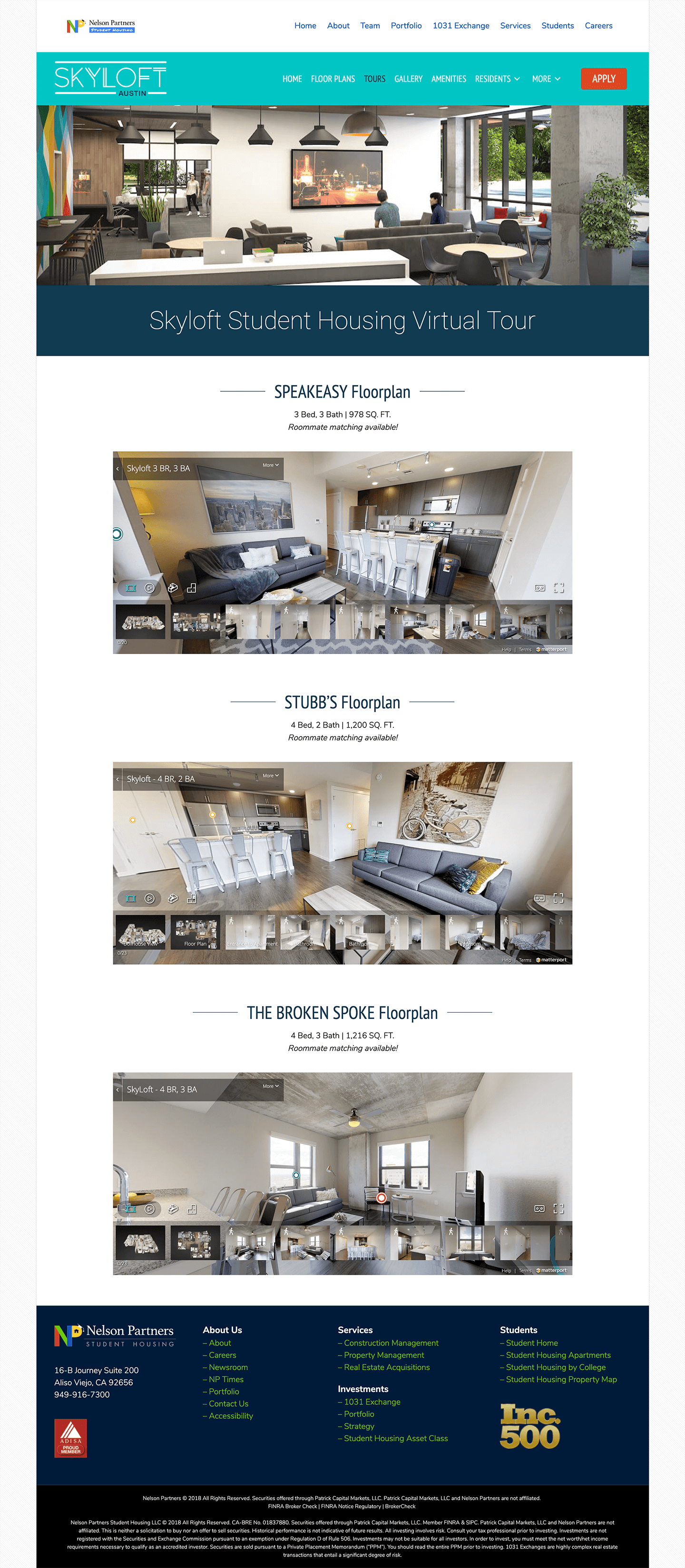**Screenshot Description of Skyloft Student Housing Virtual Tour Website on Smartphone**

This screenshot displays the mobile version of the Skyloft Student Housing Virtual Tour website, captured on a smartphone, indicated by its narrow width. 

**Header and Logo:**
- At the top-right corner, a colorful logo features a combination of red, green, blue, yellow, and black colors forming an 'N' shape.
- The primary navigation menu is aligned to the right, likely containing links to various sections of the website.

**Main Banners:**
- Below the header, there are two banners:
  - The first banner is blue with black text overlaying white text, the contents of which are illegible due to low resolution.
  - The second banner has a teal background with predominantly white text and some black text, featuring a red "Apply" button on the right side.
  - The text suggests that the website is showcasing a virtual tour of Skyloft Student Housing.

**Content Section:**
- Beneath the property-specific banner, there is a descriptive block of text titled "Skyloft Student Housing Virtual Tour."
- An image situated between the header and this text depicts a communal area, possibly featuring seating arrangements, work surfaces, a TV, artwork, and some plants. The view outside shows what seems to be a parking lot, making it hard to determine if it’s an artist's impression or a real photograph due to the resolution quality.

**Floor Plans:**
- The website showcases three different floor plans with detailed information:
  1. **Speakeasy Floor Plan**: 3-bedroom, 3-bathroom, 976 sq. ft.
  2. **Stubbs Floor Plan**: 4-bedroom, 2-bathroom, 1200 sq. ft.
  3. **Broken-Spoke Floor Plan**: 4-bedroom, 3-bathroom, 1215 sq. ft.
- Each floor plan title is in dark blue, with details such as the number of bedrooms, bathrooms, and square footage appearing beneath in a smaller, centered font. Additional italicized text is present but not legible.

**Image Gallery:**
- There is an embedded gallery displaying eight separate images with a ninth one partially out of frame, suggesting interactive features to view individual images within the space.

**Footer Section:**
- The footer contains extensive text, likely disclaimers and necessary disclosures common in real estate.
- The footer mentions "Nelson Partners Student Housing" with the logo described earlier.
  - The logo integrates an 'N' and 'P', with the 'P's bubble stemming from the 'N's upstroke, featuring red (vertical), green (angled), blue (vertical), and yellow colors.
- The footer includes the address, phone number in white, and an accreditation logo in red.
- There are several sectional links including About Us, Careers, Newsroom, Portfolio, Accessibility, Contact Us, Services, Property Management, Real Estate Acquisitions, Investments, Portfolio Strategy, Asset Class.
- In the final columns, options related to "Students" are present but the full details are difficult to read.
- The footer also displays the INC 500 logo, indicating a notable designation for the company.

This detailed description provides an overview of the elements present in the screenshot, with specific highlights on its visual structure, primary content, and footer layout.